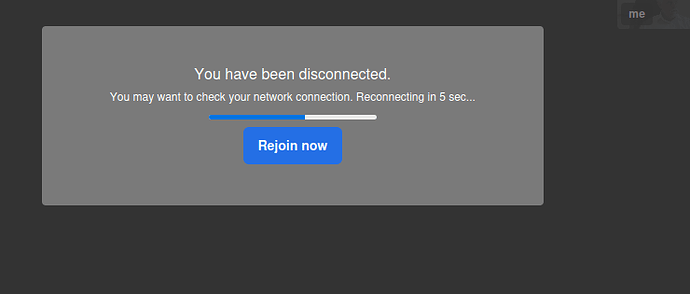The image showcases a scenario that is universally dreaded on digital screens—a disconnection notice. Dominating the display is a large gray notification box. In the top right corner of this box, there is a smaller, lighter gray rectangle featuring the text "ME" inside yet another lighter gray box.

An identical gray box appears as though it has been dragged and repositioned to the lower left corner. This box contains a white text message that reads, "You've been disconnected. You may want to check your network connection. Reconnecting in 5 seconds...". Below this message is a contrasting blue button with the text "Rejoin Now." Additionally, there is a progress bar above the button, split evenly between blue and white, likely indicating the rejoining process.

This unexpected interruption can be particularly frustrating as it disrupts ongoing activities, highlighting the importance of a stable network connection.